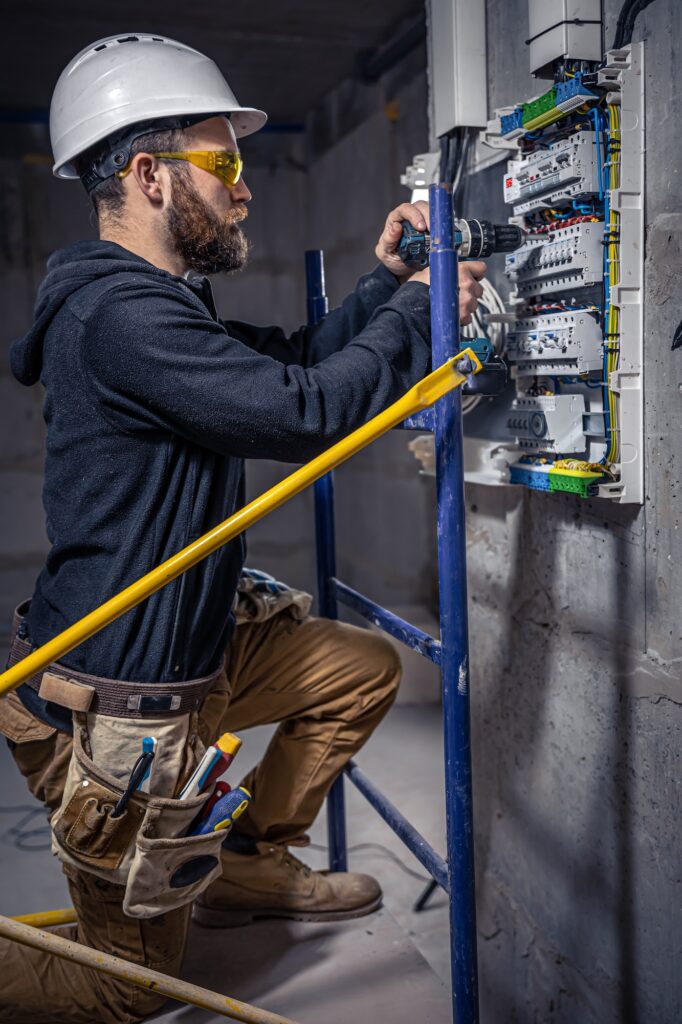The image depicts a man engaged in electrical work inside a concrete structure. He's squatting on a blue and yellow scaffolding and is focused on an open electronic panel attached to the wall. The panel contains a myriad of colored wires, including blue and red. The man is equipped with a white hard hat and yellow safety glasses, indicating a potentially hazardous environment. He wears a long-sleeved black hoodie, brown pants, and sturdy work boots. A tool belt encircles his waist, filled with various tools. He holds a drill in both hands, busily attending to the panel.